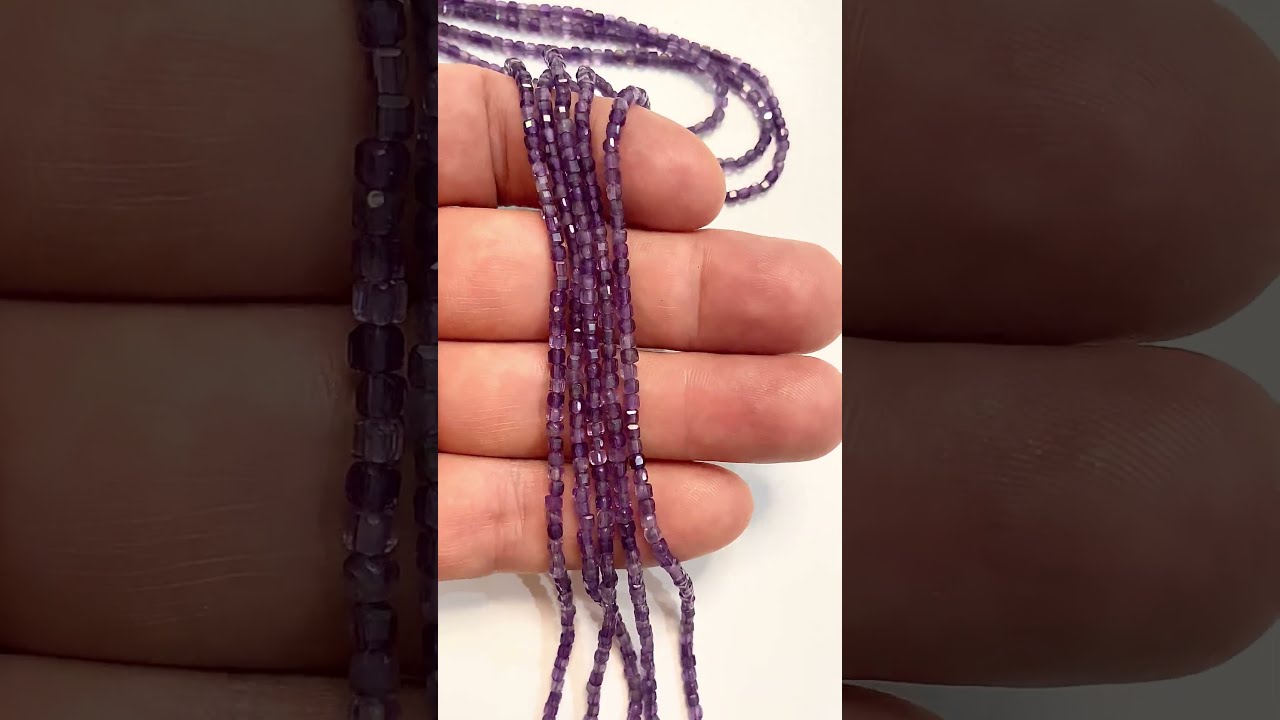The image captures a close-up view of a person's hand, resting on a flat white surface, as it holds five strands of small, cylindrical purple beads strung on thin strings. The hand, showing four fingers but not the thumb, is a light pinkish hue and displays intricate skin details such as wrinkles and fingerprints, which are subtly mirrored in the dimmed, zoomed-in borders on either side of the image. These borders, created from enlarged sections of the main picture, add depth and context to the central focus. The beads vary slightly in shape, with some appearing more square and others rounder, and exhibit a spectrum of purple shades, ranging from dark to light, with some beads seemingly translucent. The strands of beads drape over the fingers, creating a visually engaging display against the stark white background.